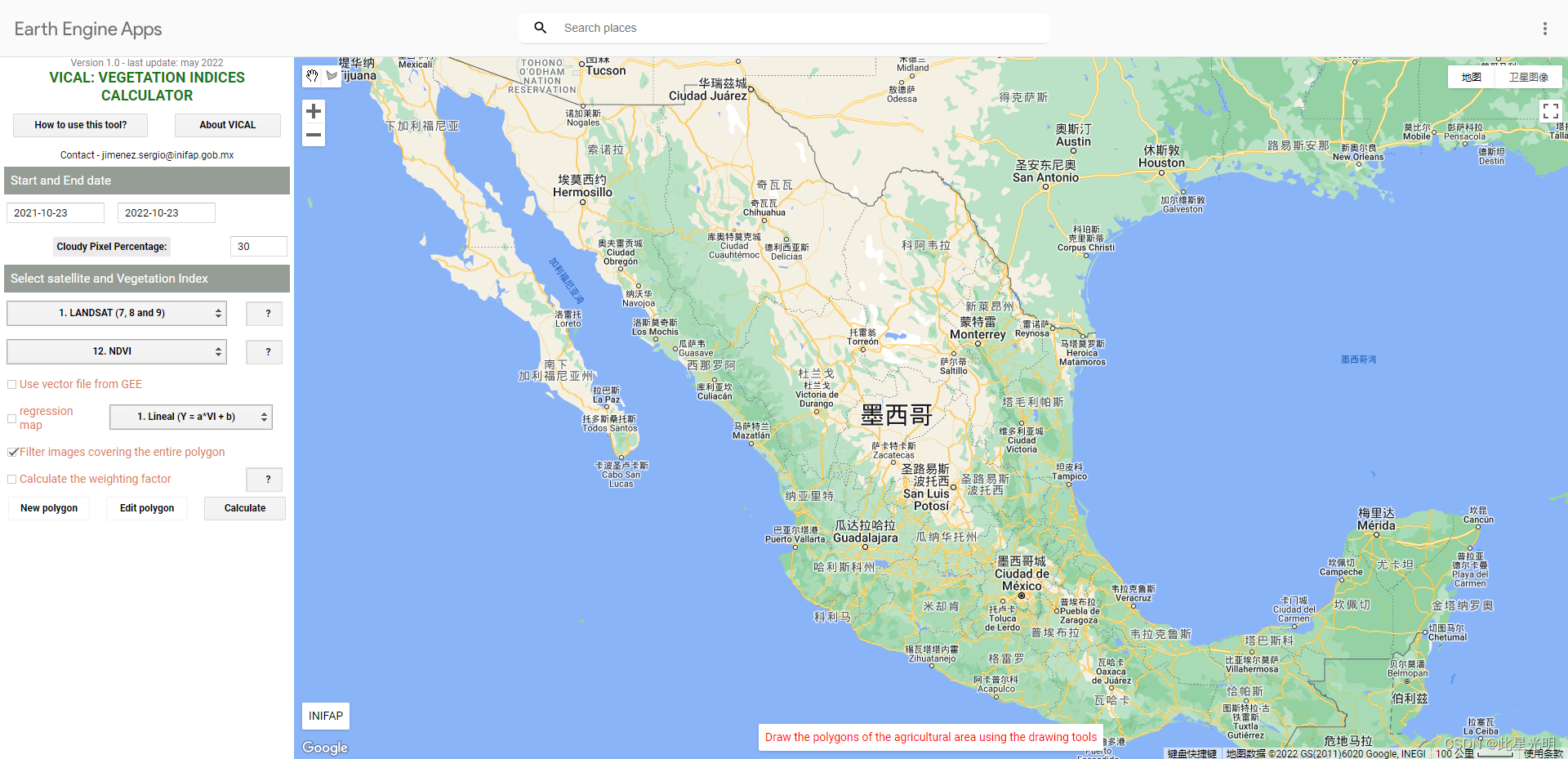This is a detailed description of a map screenshot displaying vegetation indices information. The top-left corner features the text "Perth Engine Apps," while a nearby small, hard-to-read text appears to discuss various vegetation indices calculators. The main section of the image to the right showcases a large map, predominantly labeled in Chinese. Despite the language barrier, the map outlines geographic regions starting from the United States' southern border, extending through Mexico, and covering the entirety of South America, including Brazil and its southernmost areas. The Gulf of Mexico is visible to the right of the map, and the Pacific Ocean is depicted to the left. The map thus serves as a visual representation of vegetation data overlayed with geographic and linguistic elements, suggesting its use in agriculture or environmental studies.